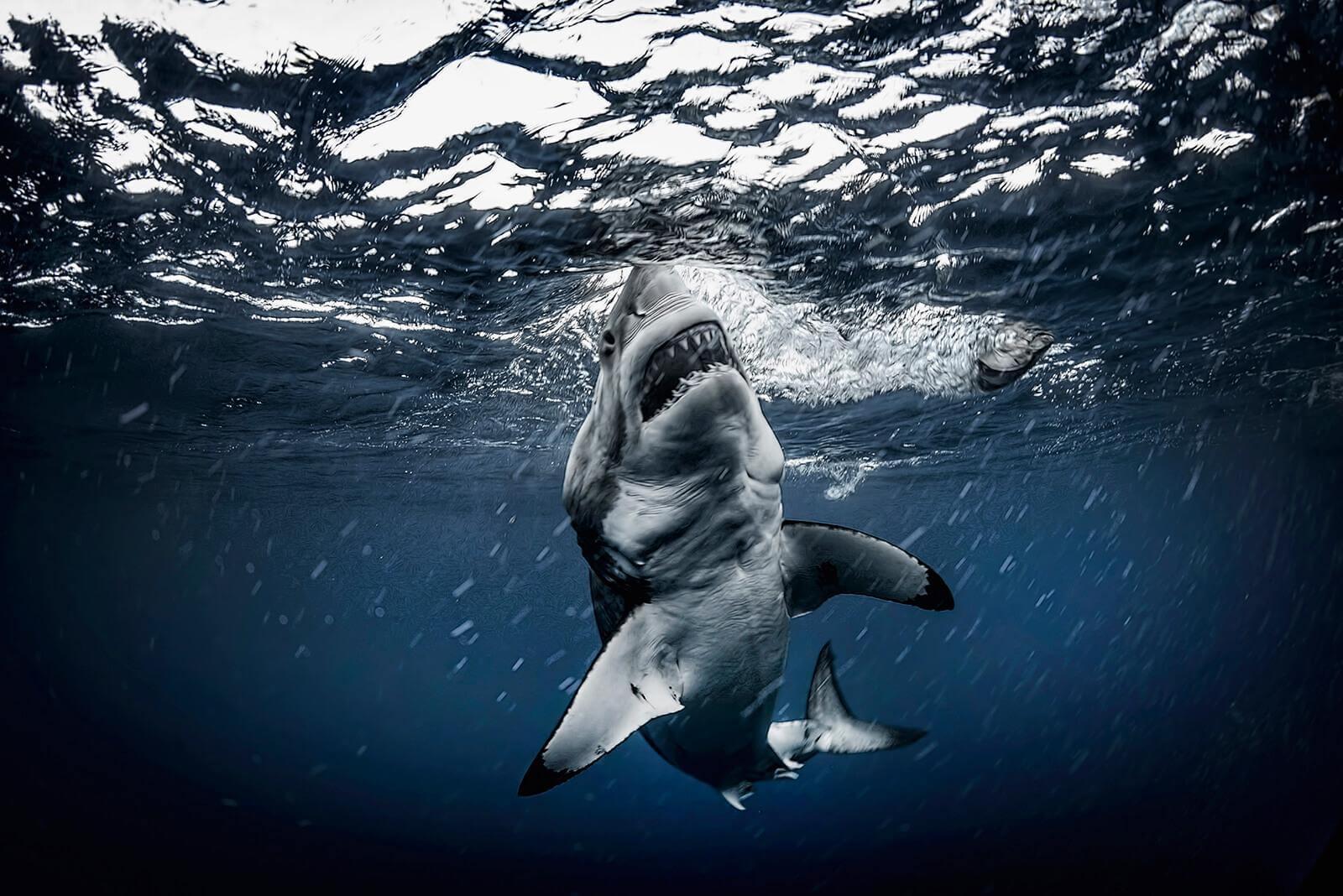The image showcases a hyper-realistic, computer-generated great white shark viewed from underneath, focusing on its muscular build and ferocious appearance. The shark, positioned with its head nearing the water's surface, displays an open mouth with sharp, prominent teeth. The scene captures the underside of the shark, highlighting its unique, weight-lifter-like musculature and the white coloration of its belly contrasted by darker edges. Disturbances in the water surround its nose and trail behind its body, with visible side fins and the tail extending far back. The top of the image reveals the water's surface, slightly blurred with raindrop-like specks pushing through, creating an impression of a recent rainfall. The ambient light, partially obstructed by waves, adds a dramatic effect, enhancing the overall intensity and realism of the photo.